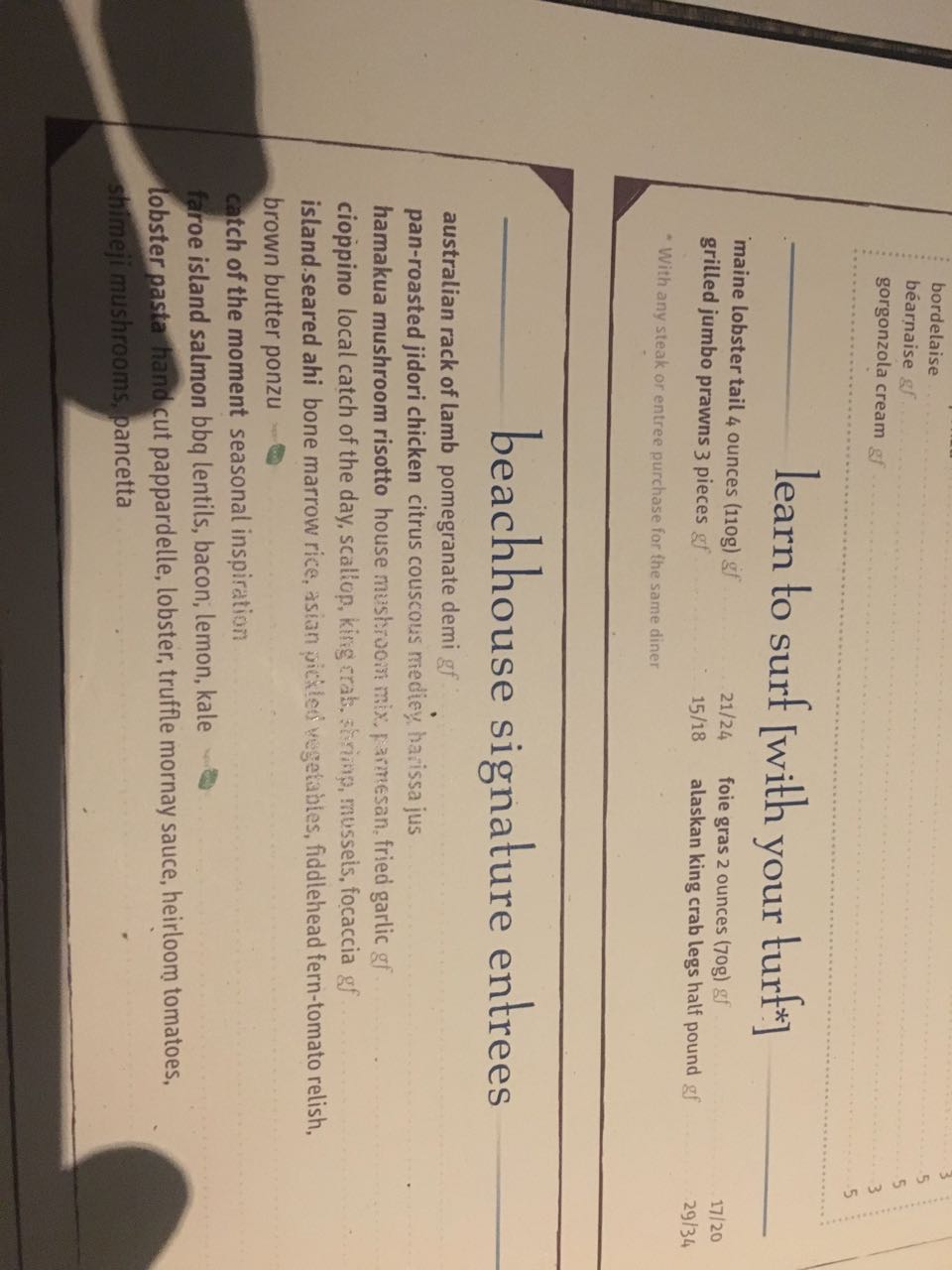**Caption:**

This color photograph, currently rotated 90 degrees clockwise, showcases a detailed menu laid out on white or off-white paper. To properly view the menu, the image should be rotated 90 degrees counterclockwise. Presently, there is a shadow cast by fingers visible at the bottom of the menu; two fingers are positioned at the current bottom-left (which will become the top-left upon rotation) and the shadow of another finger appears at the current bottom-right (which will become the bottom-left upon rotation).

The menu features an array of surf-and-turf options, suggesting it belongs to a high-end steakhouse with a seafood focus. Key items listed include "Learn to Surf with Your Turf," offering Maine Lobster Tail (4 ounces/110 grams), Grilled Jumbo Prawns (3 pieces), Foie Gras (2 ounces), and Alaskan King Crab Legs. Above this section, there are mentions of various cheeses including Gorgonzola.

Headers on the menu are printed in navy blue while the rest of the text appears in black or brown. The section titled "Beach House Signature Entrees" lists dishes such as Australian Rack of Lamb with Pomegranate Demi-Glace, Pan Roasted Jidori Chicken served with Citrus Couscous and accompanying medley, as well as Hamaku Mushroom Risotto featuring house mushroom mix, Parmesan, and fried garlic. Other standout dishes include Cioppino, packed with local catch of the day, scallop, king crab, shrimp, and mussels, served alongside focaccia.

Further down, the menu highlights Island Seared Ahi with bone marrow rice, Asian grilled vegetables, fiddlehead fern, tomato relish, and brown butter ponzu. Another intriguing entry is the "Catch of the Moment," described as a seasonal inspiration. There is mention of another dish potentially involving salmon but partially obscured by a shadow, listing ingredients like BBQ lentils, bacon, lemon, and kale. The Lobster Pasta follows, described with components such as lobster, truffle mornay sauce, and heirloom tomatoes.

Although the prices are not clearly visible, the array of gourmet offerings hints at an exclusive, expensive dining experience.